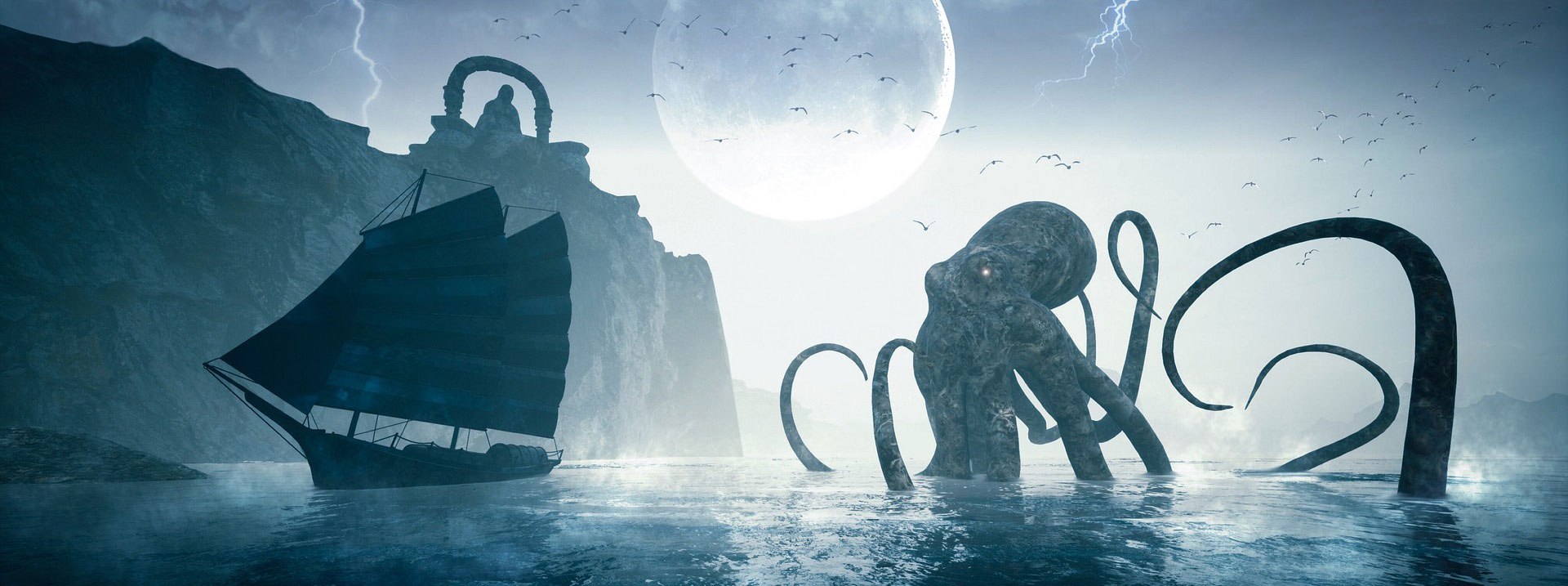This digital art piece depicts a serene nighttime ocean scene with various striking elements. Dominating the left side, towering rocky cliffs are home to a Buddha statue perched on the edge, adding a sense of mysticism. In front of the cliffs, an Asian-inspired sailing ship with distinct fan-like sails navigates the calm waters. The center of the image showcases a luminous full moon, nearly white and surrounded by bolts of lightning that starkly illuminate the dark sky. Adding a dramatic and mythical touch to the scene, a colossal octopus-like creature, reminiscent of Cthulhu, emerges from the water, its menacing tentacles partly submerged yet poised towards the sailing ship. Birds in flight enhance the depth of this computer-generated art, which is beautifully rendered in shades of blue, white, and black.